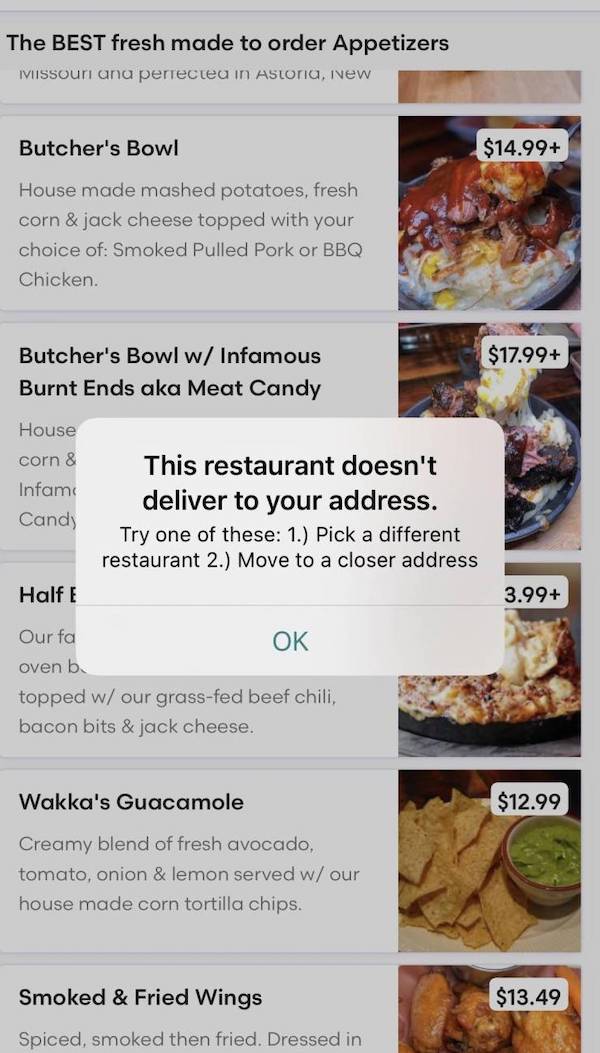This screen capture is taken from a food delivery website, possibly resembling Grubhub. The image features a pop-up window overlay informing the user that the selected restaurant does not deliver to their address. The message offers two suggestions: "1. Pick a different restaurant" and "2. Move to a closer address," followed by an "OK" link below.

In the background, the website displays a menu with a series of rectangular blocks, each providing detailed information about various food items. The layout includes:

1. The top block featuring the "Butcher's Bowl," described as house-made mashed potatoes, fresh corn, and cheese topped with a choice of smoked pulled pork or barbecue chicken. Adjacent to this description is a photograph of the dish with an overlay displaying the price, $14.99, in a white rectangular box with black lettering.
2. The next block presents the "Butcher's Bowl with Infamous Burnt Ends," also referred to as "meat candy."
3. The final block at the bottom highlights "Waka's Guacamole."

Each item follows a similar format: the name and detailed description of the dish on the left, a photograph of the food on the right, with the price clearly indicated in an overlay on the image. This thorough layout suggests that the website aims to provide comprehensive information to help users make informed decisions about their food orders.